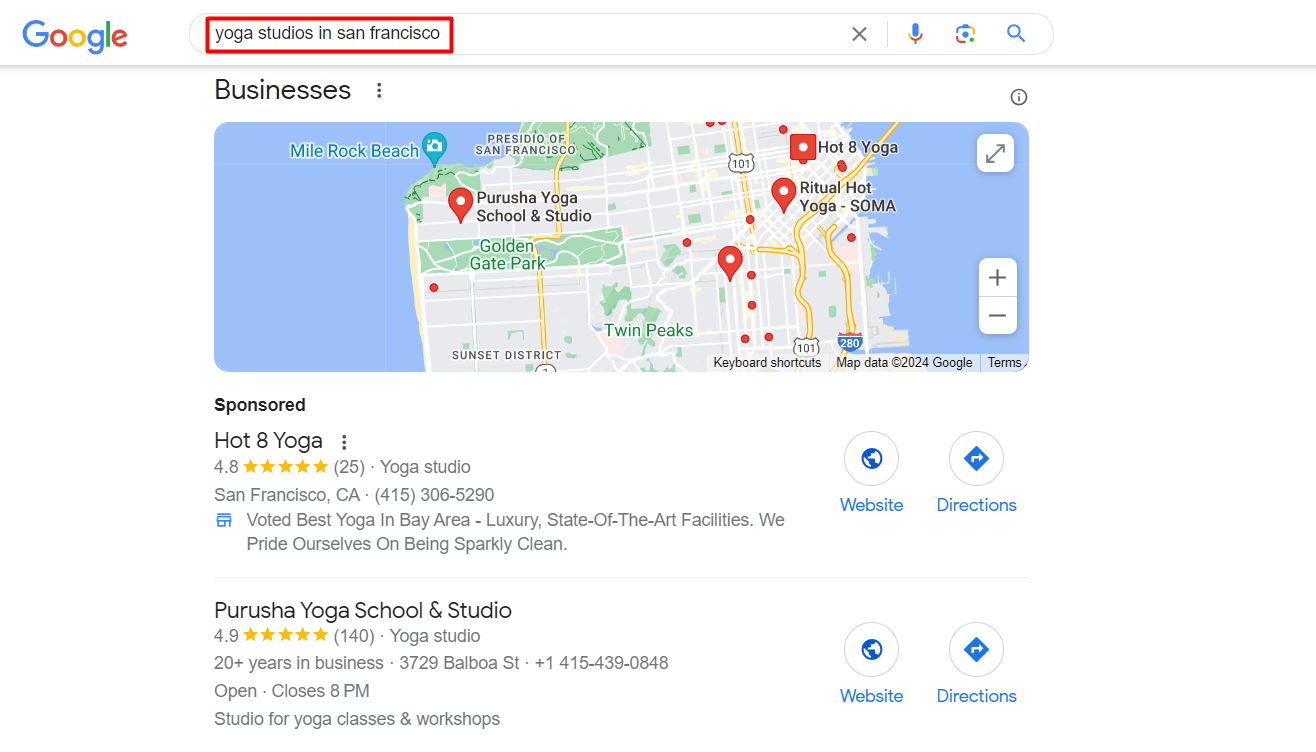The image is a Google Maps search result showing yoga studios in San Francisco. The map highlights a narrow strip of land, flanked by water on both sides, notably featuring Mile Rock Beach. Notable points of interest in the vicinity are illustrated, including the Presidio San Francisco, Golden Gate Park, and the Sunset District.

The search results display two yoga studios prominently. The first listing, Hot 8 Yoga, is a sponsored advertisement boasting a 4.8-star rating out of 5 from 25 reviews. It is described as the best yoga studio in the Bay Area, offering luxury, state-of-the-art facilities, and emphasizing a pristine, sparkly clean environment.

The second listing, Purusha Yoga School and Studio, is an unsponsored entry with a 4.9-star rating from 140 reviews. Unlike Hot 8 Yoga, Purusha focuses on providing a plain and simple studio for yoga classes and workshops.

Additionally, another yoga studio, Ritual Hot Yoga Soma, is marked on the map. Both listings are set against a white background, providing clear visibility of their descriptions and ratings.